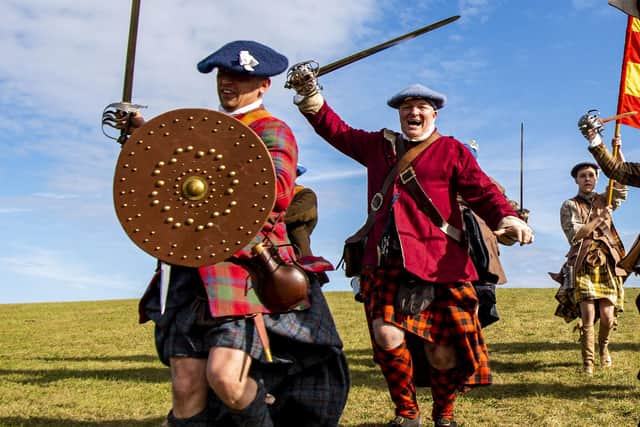In a vibrant outdoor scene under a bright blue sky with scattered clouds, a vivid portrayal of historical reenactors unfolds on a lush green grass field. Dominating the foreground is a man clad in a traditional kilt paired with a plaid shirt and a blue hat, holding a sword in his right hand and a circular shield in his left. His kilt, exhibiting intricate patterns, sways as he moves, casting shadows that hint at the sunny day. Right behind him stands another man, dressed in a gray hat, red jacket, and a plaid kilt matched with high plaid socks. This second man, equipped with a sword held firmly in his right hand, strikes a dynamic pose. Further back, a figure, likely a woman based on her attire, is garbed in a light tan plaid skirt and holds a partially visible red and yellow flag. Additional indistinct forms of people frame the trio, reinforcing the lively atmosphere. The entire scene is devoid of trees, emphasizing the human elements and their period attire, evocative of the 17th or 18th century. The combination of swords, kilts, and vibrant clothing infuses the image with historical richness and action, capturing a moment frozen in time.